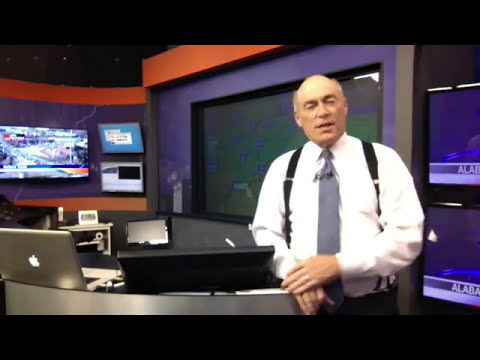The photograph is a square, color image framed by thick black borders at the top and bottom, capturing the scene of a bustling newsroom. Dominating the right side of the image, a man in his 60s with slight gray hair on the sides, bald atop, looks directly at the camera with squinted eyes and an open mouth, appearing to speak to the viewer. He is dressed in a long-sleeved white button-down shirt with a gray tie showing a hint of blue, and black suspenders. Leaning on a chrome-topped desk, he has his arms crossed in front of him. The desk is cluttered with tech devices, including an open silver Apple laptop and an adjacent black monitor. Behind him, a large screen displays a map, suggesting he may be delivering a weather or traffic report. Further back, to the left, another TV screen and two more monitors are mounted on the wall, broadcasting additional content. To the right edge of the frame, the phrase "Alabama" is visible on the screen of one of two more monitors. The background features walls with alternating purple and orange hues, contributing to the high-tech, dynamic atmosphere of a modern broadcast studio.